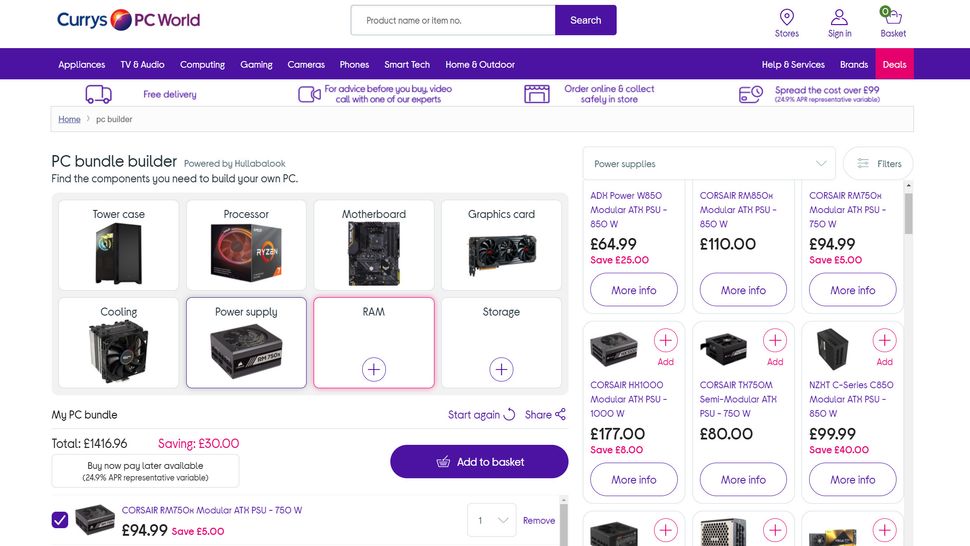The screenshot shows the PC World online store interface, specifically the PC bundle builder section. At the center, there's a prominent image of a tower case alongside components like graphics cards and a motherboard. The top of the page features a purple navigation bar with options for "Store," "Sign In," and "Basket." Below this bar, there's a pink square highlighting special deals. A search bar is available for users to find specific items, and to the right, a list of around eight power supplies can be scrolled through. 

In the lower section of the screen, there is an option to review "My PC Bundle," which allows users to see their selected components. The buttons associated with this feature have white backgrounds with purple text. Additionally, pink writing in the interface indicates potential savings, providing a clear and informative shopping experience.